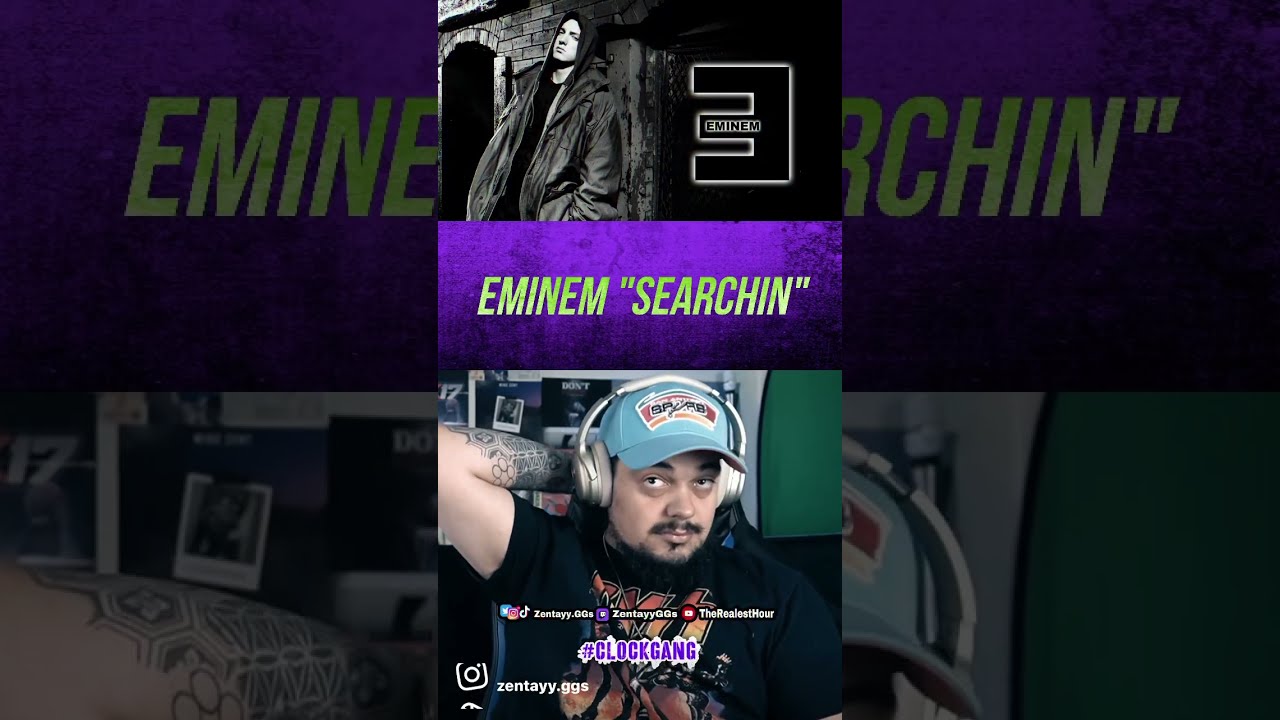The image appears to be a screenshot from a video, divided into three main sections. The top section features Eminem leaning against a wall with a stylized logo, including a backwards 'E' and the name "Eminem" outlined in white. The middle section prominently displays the text "M&M Searchin'" in a yellowish-green font on a black background. The bottom section showcases a man who looks like a DJ, wearing a light blue Spurs cap and silver headphones with one arm bent behind his head. He's dressed in a black shirt with the word "Kiss" on it, set against an orange background. His right arm has a noticeable tattoo. The background and sides of the image have a mix of colors, including light blue, green, silver, black, orange, purple, and white. The overall layout resembles a TikTok or social media video screenshot, featuring different hashtags and usernames, such as "#clockgang" and "zente.ggs".